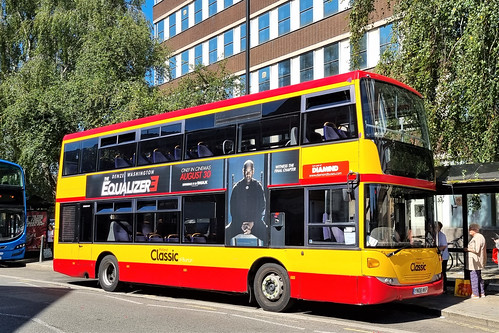This photo features a classic double-decker bus prominently situated in the foreground, adorned in bright red and yellow colors. The bus has large windows on both levels, providing a clear view of the seating inside. Notably, a distinct yellow stripe runs down the length of the bus, accentuating the middle section below the seating area.

A striking advertisement for the movie "The Equalizer 3" with Denzel Washington is displayed in the center of the bus. The ad, which features the actor sitting on a chair and staring intently at the camera, promotes the film's release date of August 30th. Washington is dressed in all black and is backlit, making his image particularly striking against the bus's vibrant background.

The scene captures the bus at a city bus stop, ready to pick up passengers. A woman in blue jeans and a beige shirt stands next to the bus, seemingly engaged at a ticket booth. Another person is also visible nearby, contributing to the bustling urban atmosphere.

In the background, the cityscape features a tall building with numerous windows and large trees with abundant green foliage. The front of a blue bus is partially visible behind the red and yellow double-decker, adding to the depth and context of the urban setting.